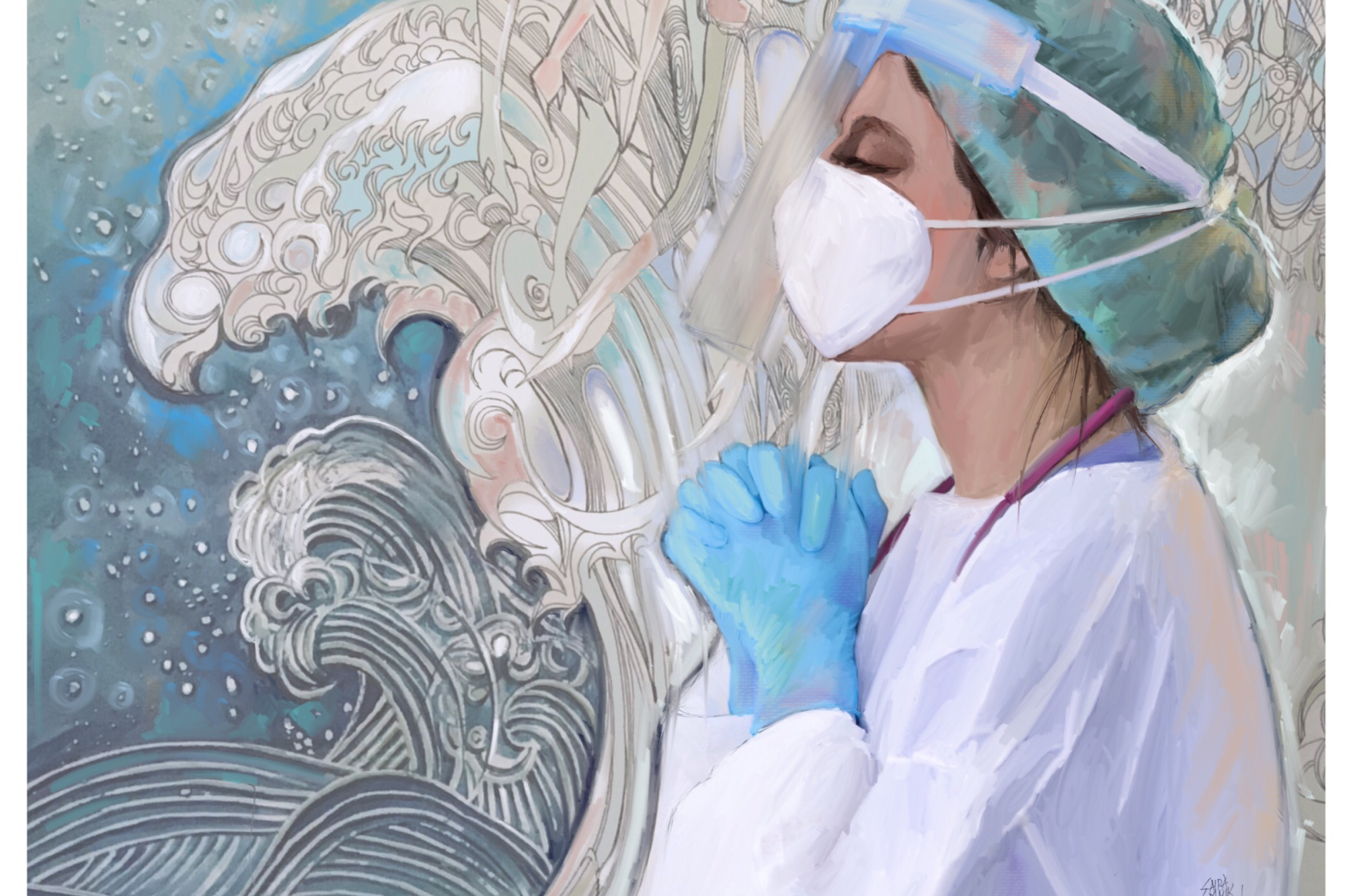This work of art depicts a young female nurse in full operating room attire, captured in a moment of prayer. She is shown in profile, facing left, with her hands elevated and clasped in front of her chest, eyes gently closed. The nurse is adorned in a surgical cap, face mask, a protective plastic shield, blue surgical gloves, and a white smock. Behind her unfolds an intricate background of ocean waves. A prominent wave, depicted in various shades of light blue and white with elaborate, curly shapes, stands out. Beyond this, the backdrop transitions to a darker blue ocean with waves outlined in white. The waves seem almost to emanate from her presence, adding a sense of depth and connection between the nurse's serene moment of prayer and the natural, powerful beauty of the ocean.